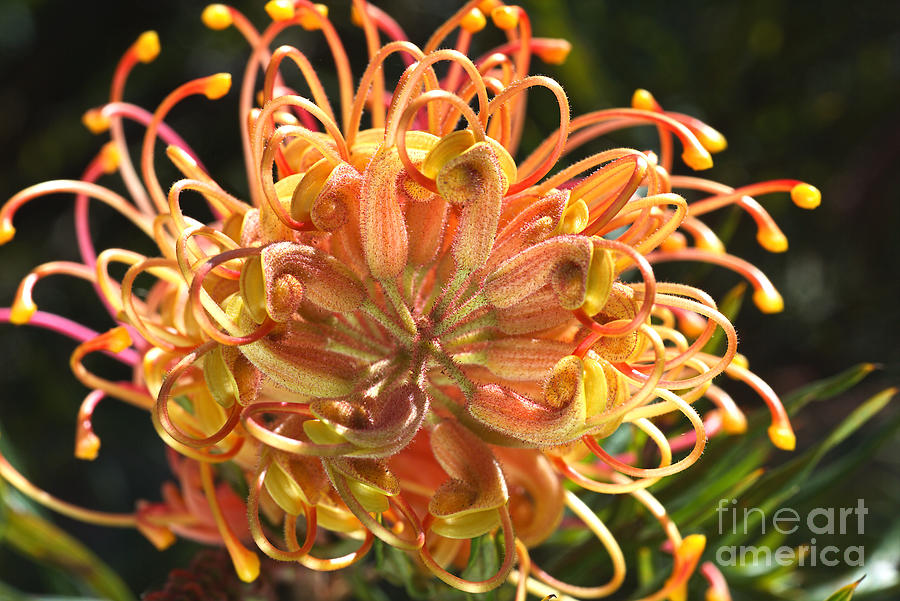The image is a professional, close-up photograph of a strikingly beautiful flower, prominently featuring the flower's head in vivid detail. The background is a lush, blurred green, providing a soft, unobtrusive contrast that highlights the flower. The flower showcases a mesmerizing blend of colors, including vibrant shades of orange, yellow, reds, and hints of pink. It appears adorned with long, thin, leggy stamens, each tipped with yellow, adding intricate detail to its overall appearance. The petals reveal a rich, colorful mix of pink, yellow, and red, making the floral display exceptionally eye-catching. At the bottom right corner of the image, the text "Fine Art America" is subtly embedded, suggesting the image's professional quality. The sunlit day enhances the flower’s natural beauty, with soft sunlight casting a glow on the petals, bringing forth the full splendor of the close-up composition.